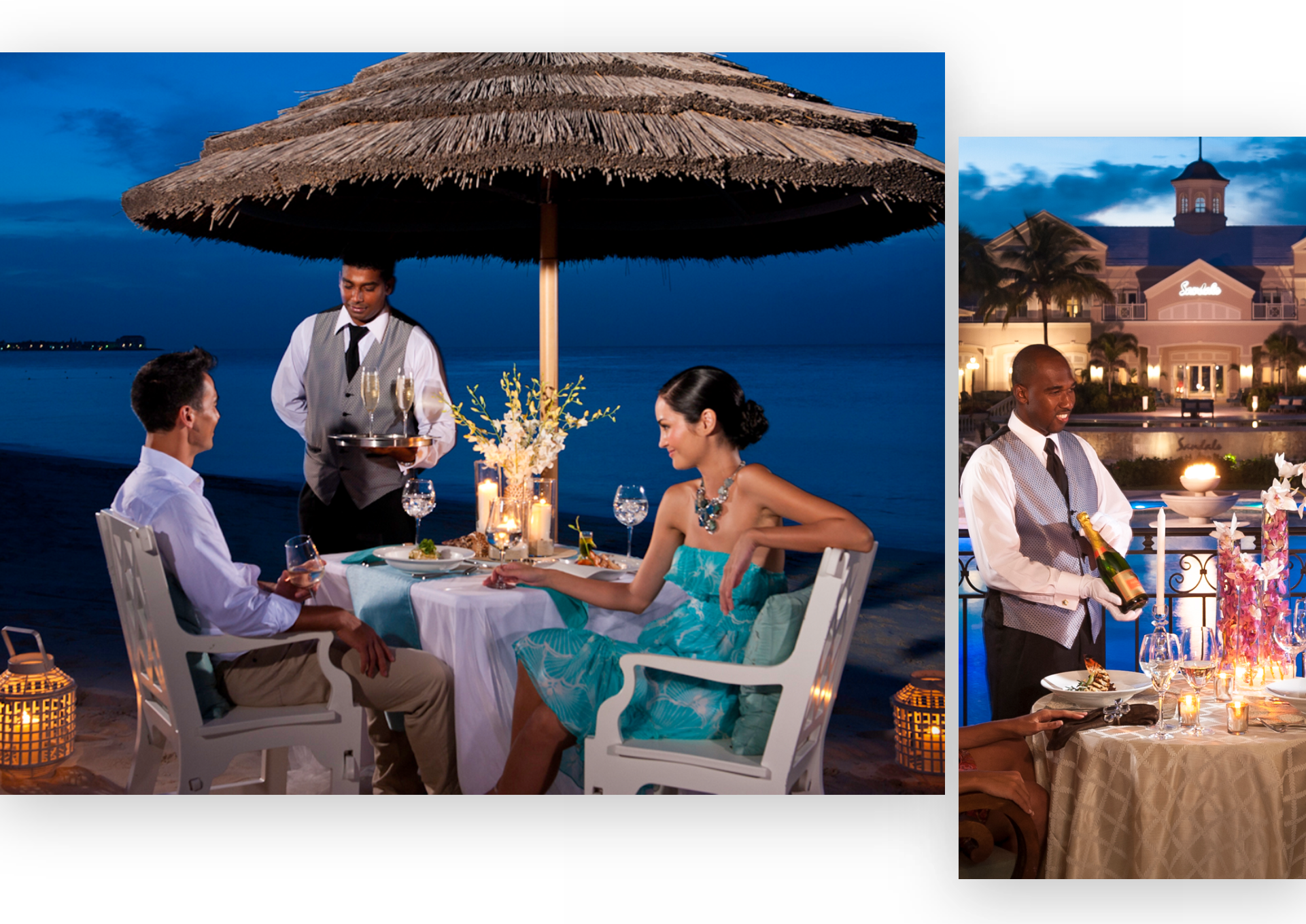The image features two photographs placed side by side, exemplifying an elegant, tropical-themed resort, possibly Sandals. The larger left-hand photograph captures an idyllic evening scene with a couple dining al fresco by the ocean, under a thatched tiki umbrella. They are seated on intricately carved white chairs, an African-American waiter elegantly dressed in a white shirt, silver vest, and black tie serves them champagne in fluted glasses. The table, adorned with a white tablecloth, turquoise napkins, flowers, and two lit candles, adds to the romantic atmosphere. The woman in a turquoise and white halter dress with a silver and blue necklace complements the décor, while the man, dressed in a light blue shirt and khaki pants, looks equally relaxed. The background reveals a vast body of water with city lights twinkling in the distance. 

The smaller right-hand photograph depicts a similar but more distant scene. Another African-American server dressed in the same attire presents a bottle of champagne to an out-of-frame couple. The table setup is equally elegant with white dishes, crystal glasses, and two tall candles, situated near a lit-up hotel identified as "Sandals," accompanied by towering palm trees in the background. A body of water also features in this photo, suggesting a pond facing the hotel, contrasting the ocean view in the left photograph.